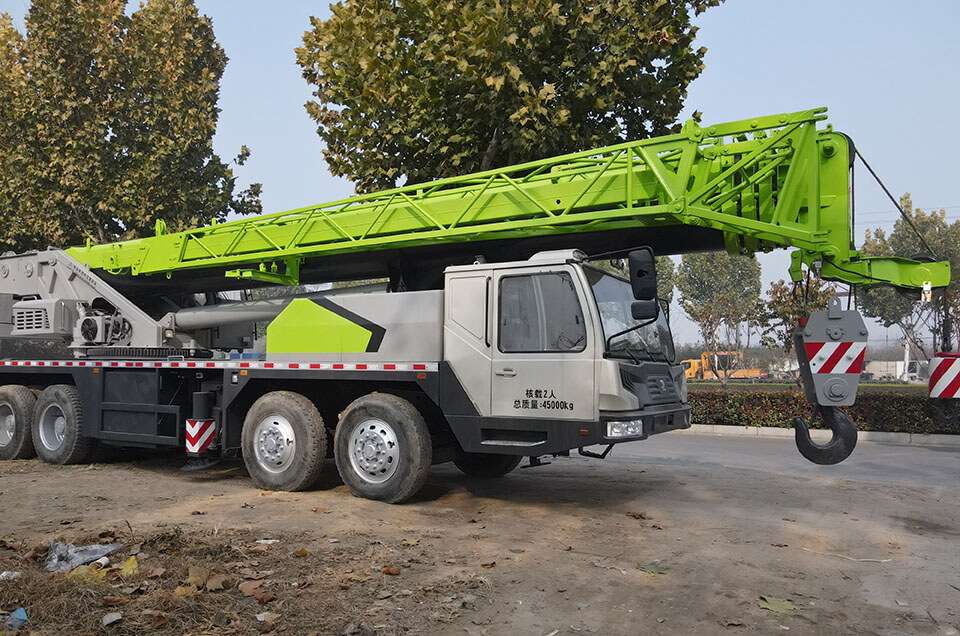This photograph showcases a large, gray construction truck featuring an extensive crane mounted on its chassis. The crane, most notably characterized by its vibrant lime green hue, lies flat atop the truck with a hefty hook dangling from it, adorned with red and white stripes at its base. The truck, which bears eight wheels, is marked with Asian characters, suggesting it is located in an Asian country. Surrounding the truck is a predominantly muddy brown ground, scattered with dying leaves. The background reveals a clear, semi-blue sky with several fully-leaved trees—two prominent ones in the foreground and four more distant ones. Additionally, a red and white traffic cone is positioned to the right side of the image, indicating an active construction site.